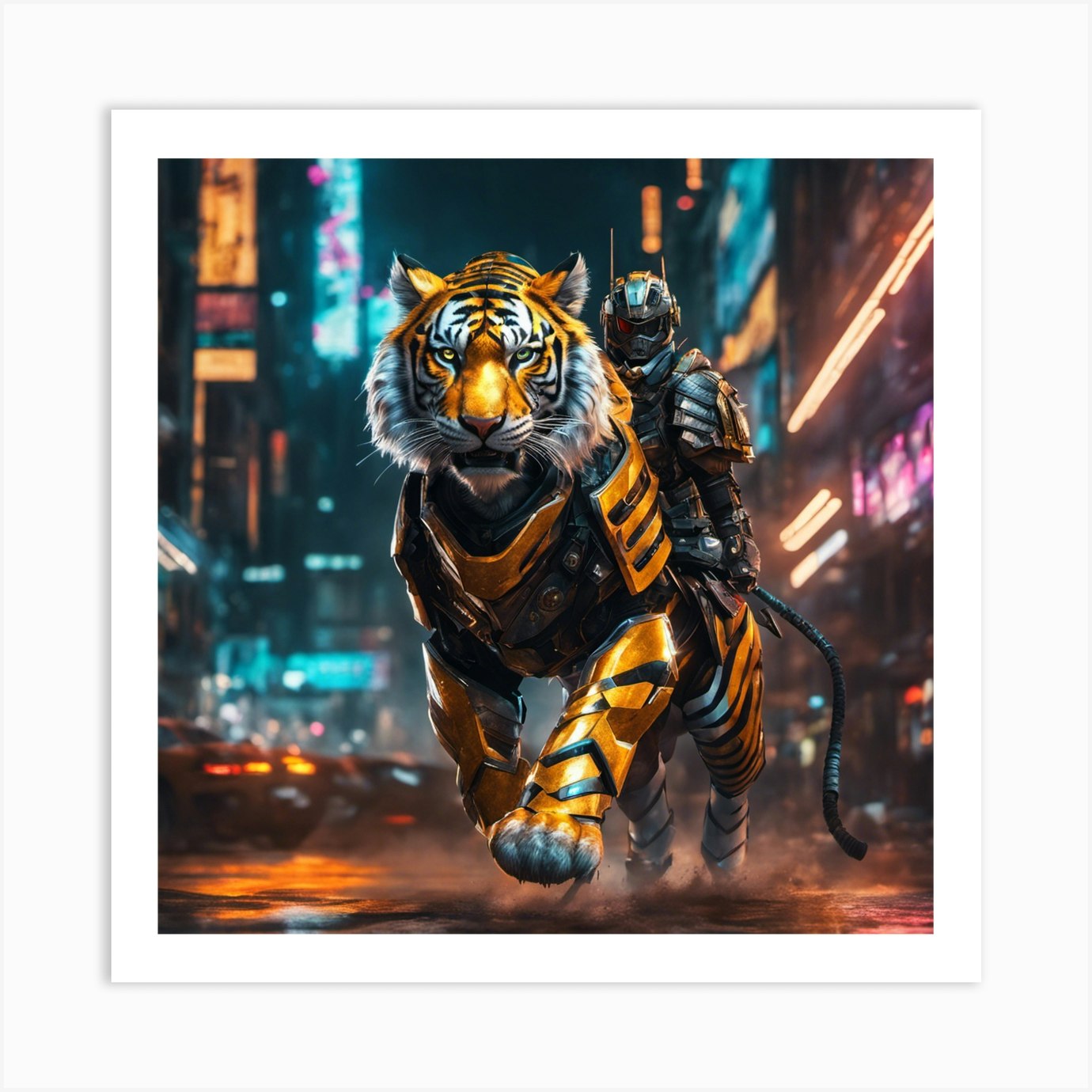The image depicts a vividly detailed graphic art scene featuring a highly stylized, robotic tiger in motion. The tiger combines organic and mechanical elements, with a head adorned in traditional orange fur, black stripes, and realistic whiskers, while its body boasts intricate orange and black striped metal armor. The tail is a digital electric extension adding to its futuristic appearance. It is dashing through an urban setting reminiscent of a modern-day city, possibly Tokyo, characterized by towering skyscrapers, neon lights, and blurred, out-of-focus buildings. Alongside the metallic tiger, there is a robotic individual—potentially a superhero or villain—clad in ominous black armor and a helmet, sitting behind the tiger as it navigates the city. The scene is dynamic and charged with a blend of science fiction and fantasy elements, essentially capturing a moment of intense action within a bustling metropolitan landscape.